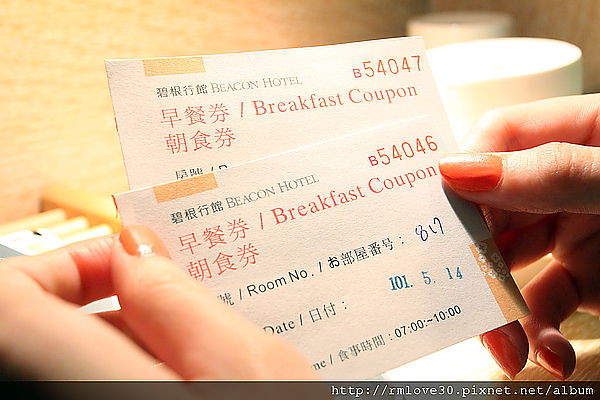This is a detailed picture of a woman holding two breakfast coupons from the Beacon Hotel. Both her left and right hands are visible, showcasing her orange nail polish. The coupons, which are identical and staggered to show both their numbers, are numbered B54047 and B54046 in the upper right corner. The coupons are printed in white and have various Chinese symbols on them. The name "Beacon Hotel" is situated in the upper left corner in red, followed by Chinese writing below.

Each coupon includes a room number and a date, with oriental characters indicating the date details, and a validation time from 7 a.m. to 10 a.m. in Chinese figures. Towards the bottom right of the coupons is a stamp. Partially visible in the upper right corner of the image are two white coffee cups, hinting at a breakfast setting. The background possibly shows a hotel bed or lamp, indicating that the photo was taken in a hotel room. The image includes a hypertext link at the bottom, rmlove30.pixnat.net/album, suggesting it was sourced from an online album.